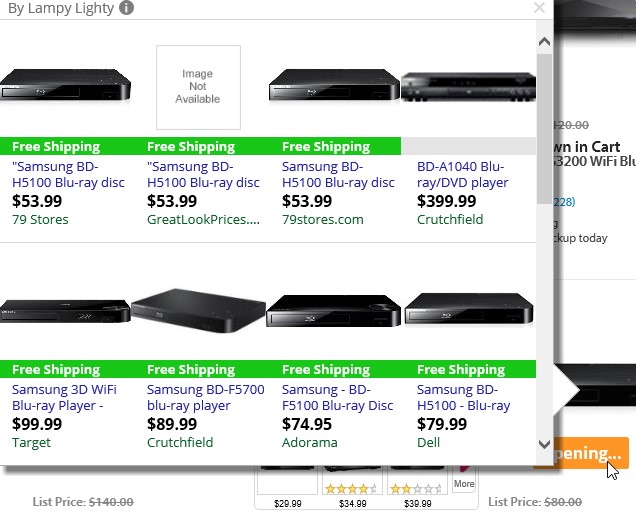Here is a detailed and cleaned-up caption based on the description provided:

---

In a horizontally rectangular image frame, a pop-up window from a retail website is displayed. At the top left corner, the header reads "by Lampy Lighty" accompanied by an information icon. Below the header, the window is organized into two rows, each containing four Blu-ray disc players. For seven of these players, an image of the device is clearly visible. Underneath these images, a green banner indicating "Free Shipping" is present for seven of the eight players. Each Blu-ray disc player listing includes the brand and model number, followed by the price and the specific store where the item can be purchased.